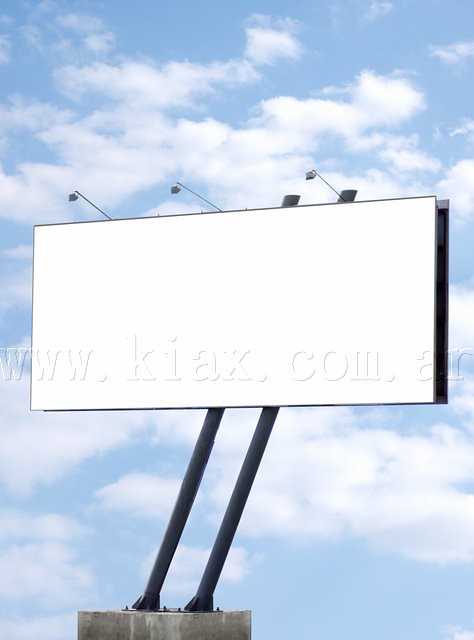In this outdoor scene, a vast and expansive sky dominates the background, painted a rich blue and adorned with numerous fluffy white clouds scattered across the horizon. At the bottom of the image, there is a concrete stand from which emerge two sturdy black metal poles. These poles support a large, blank billboard, possibly designed to be electronic, awaiting display content. Overhanging the billboard are three black lights, presumably intended to illuminate the sign during different times of the day or night. Above the billboard, a small text reads "www.kayax.com," marking the copyright for the image. The contrast between the industrial elements at the base and the natural, cloud-filled sky creates an interesting visual juxtaposition.